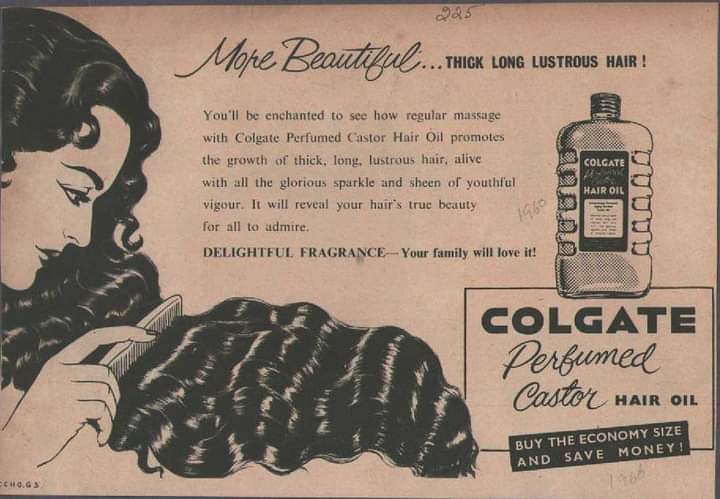The image is a vintage advertisement, likely from a magazine, showcasing "Colgate Perfumed Castor Hair Oil." The ad is in black and white, printed on what appears to be aged, beige paper. Prominently on the left side, there's a large illustration of a cartoon woman with very long, wavy black hair, which she is combing. The hair is described as thick, long, and lustrous. At the top, the number "225" is penciled in, and to the left of the bottle illustration, "1960" is also written in pencil, possibly denoting a date.

The advertisement text reads: "More beautiful, thick, long, lustrous hair. You'll be enchanted to see how regular massage with Colgate Perfumed Castor Hair Oil promotes the growth of thick, long, lustrous hair, alive with all the glorious sparkle and sheen of youthful vigor. It will reveal your hair's true beauty for all to admire. Delightful fragrance, your family will love it."

On the bottom right side, there's a drawing of a tall, upright bottle with a screw cap, labeled "Colgate Hair Oil." The bottle design appears to have ridges for easy handling. Below the bottle, the text reads: "Colgate Perfumed Castor Hair Oil. Buy the economy size and save money."